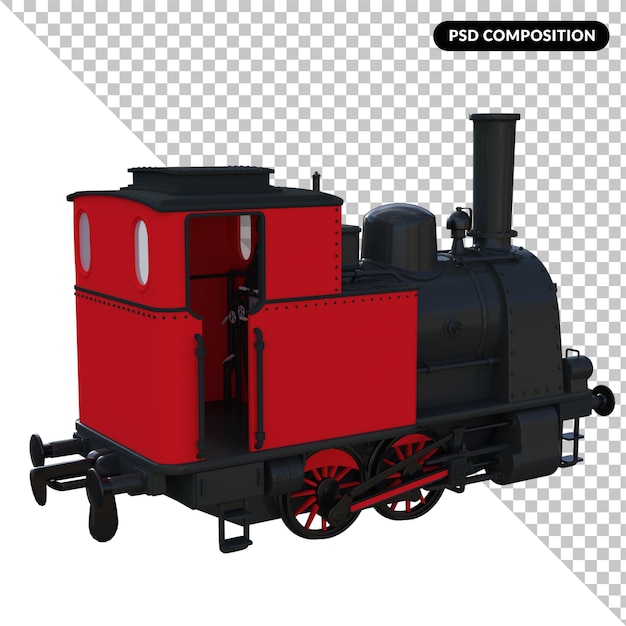The image is a detailed 3D render of an early steam engine train, labeled in the top right with "PSD Composition" within a black border with white text. The background is divided diagonally; the bottom-left half is solid white, while the upper-right half features a gray-and-white checkerboard pattern indicating transparency. The train, depicted in isolation, features a prominent black engine compartment with a red operator's section. The wheels are predominantly black with subtle red accents. The overall aesthetic suggests a late 1800s design, and the realistic yet miniature appearance hints at it being a model. This composition emphasizes the notion of the train transitioning from a solid background into a transparent one, enhancing its 3D effect.